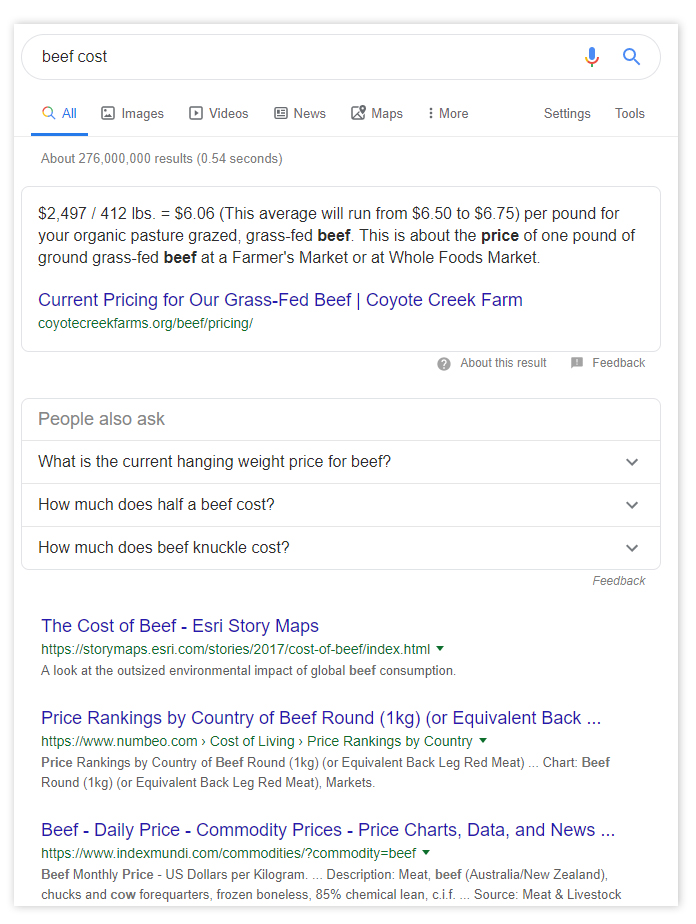The image depicts a Google search results page with the query "beef cost" entered into the search bar. At the top of the page, there is a search bar containing the phrase "beef cost," accompanied by a microphone icon and a magnifying glass icon on the right side. Just below the search bar, there are various tab options including "All" (which is currently selected), "Images," "Videos," "News," "Maps," and "More," each with corresponding icons. Additional options such as "Settings" and "Tools" are also available.

The search results return approximately 276 million entries in 0.54 seconds. The foremost result is a detailed cost breakdown, mentioning that 2,497 pounds out of 4.12 pounds equals $6.06, further explaining that the average price of grass-fed, organic pasture-grazed beef ranges from $6.50 to $6.75 per pound. It highlights that this is a typical price for one pound of ground grass-fed beef at a farmer's market or Whole Foods market. The result also references pricing information for Coyote Creek Farm's grass-fed beef.

Additionally, the "People Also Ask" section includes questions about the current hanging weight price for beef, the cost of half a beef, and the price of beef knuckle.

Several search results are listed below, featuring titles in blue such as "The Cost of Beef: S3 Story Maps - Price Rankings by Country of Beef (Round, One Kilogram or Equivalent)" and "Beef Daily Price: Commodity Prices, Price Charts, Data, and News." Each result is supplemented with a brief descriptive paragraph.